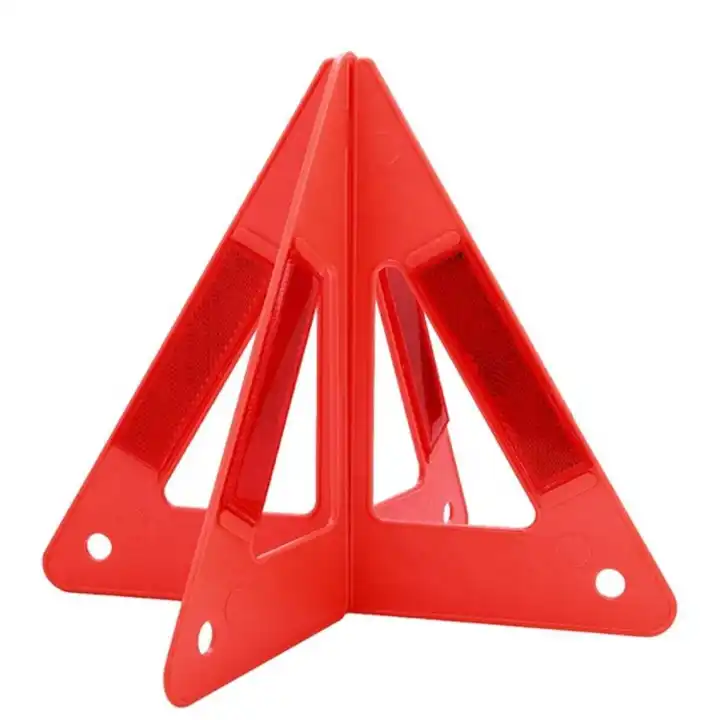The image features a cone-like structure made up of four intersecting right-angled triangles, composed of bright orange or red plastic material. Each triangle converges at a central point at the top, creating a geometric and symmetrical appearance against a white background. The triangles each have a smaller triangular cut-out near the bottom right corner and are accented with dark, rectangular reflective strips in the middle. These strips give the appearance of dark red lights. The tip and bottom base of each triangle are lighter in color, contributing to the overall visual contrast of the object. The object resembles a reflector often seen on streets and has a functional yet visually striking design.